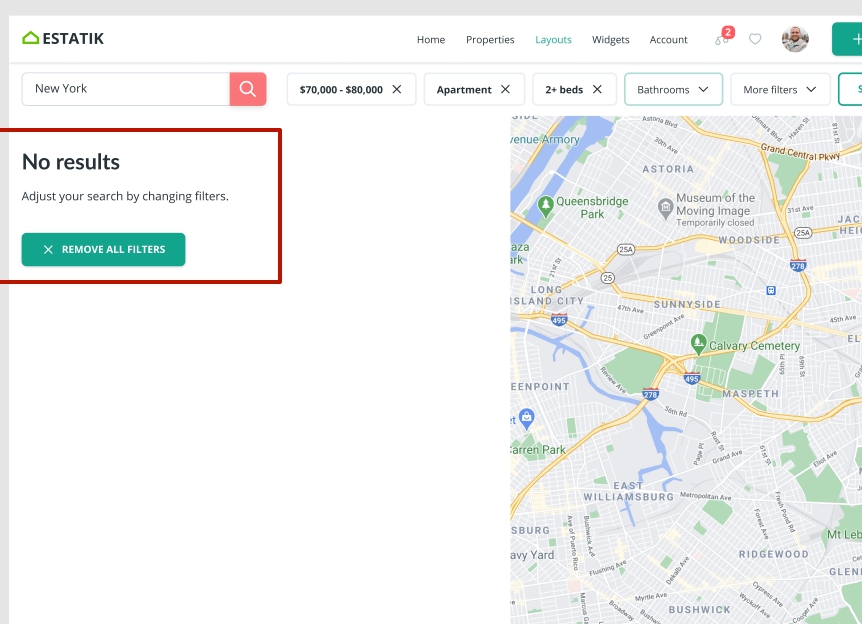**Screenshot Description: Real Estate Search on Aesthetic Website**

This screenshot captures the home page of the "Aesthetic" website, indicated by the black lettering "Aesthetic" in the top left corner, paired with a green silhouette house emblem serving as the icon. The website features a conventional navigation bar at the top, listing options such as "Home," "Properties," "Layouts" (which is highlighted), "Widgets," and "Account." Additionally, there is a notification icon with two alerts and a like symbol. It appears to be a personalized page, as evidenced by a user profile picture. 

On the far right of the navigation bar, there is a green box with a plus sign, suggesting additional options. Below this, a search bar is prominently displayed, where users can type in a location and initiate a search using a red button with a magnifying glass icon. In this screenshot, "New York" has been entered into the search bar.

Beneath the search bar, there are filter options for refining the property search. The current filters applied include a price range of $70,000 to $80,000, selection of "apartment," and a requirement of "two plus bedrooms." There are also options for specifying the number of bathrooms and more filters available for selection. The search results indicate no matches based on the current filters, prompting the user to "remove all filters and start over."

To the right side of the screen, a map of a section of New York is displayed, potentially illustrating neighborhoods like East Williamsburg, Ridgewood, Bushwick, and Long Island City. Various interstate highways and other points of interest are also visible. The precise location, possibly Brooklyn, is not clearly identifiable within the screenshot.